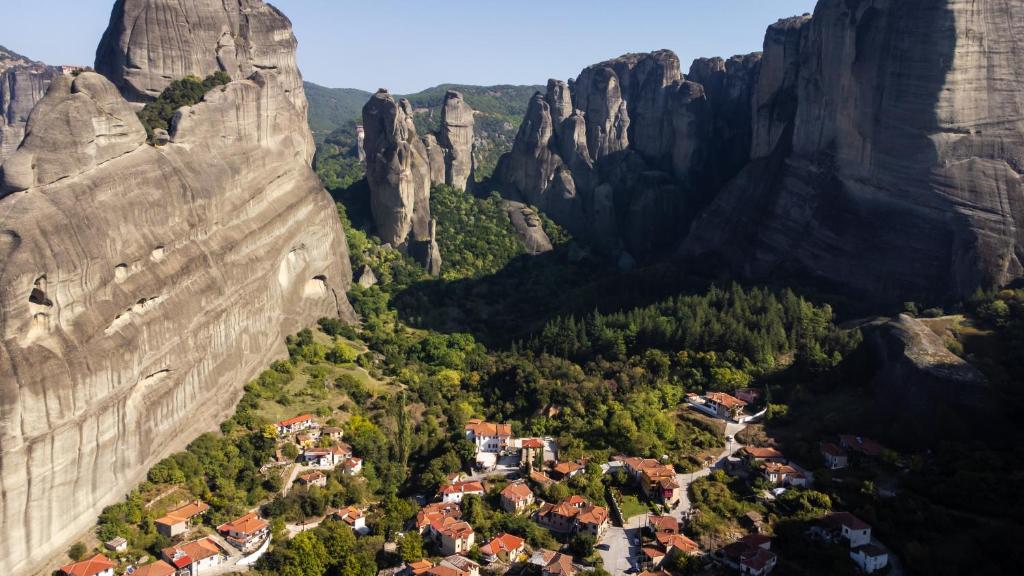This high-definition image showcases a picturesque village nestled within a forested valley, surrounded by towering stone mountain structures. The village, medium in size, is characterized by its white buildings adorned with orange-brown clay roofs, which are evident across the entire settlement. The stone mountains on either side of the image, as well as those sporadically placed in the center, are imposing and grayish in color, creating a dramatic backdrop against the vivid blue sky. The village itself is immersed in lush greenery, with various types of trees filling the spaces between the rocky formations and houses. Road structures weave through the village, possibly with a few cars navigating them, giving a sense of a serene, yet lively, environment. This amalgamation of nature and human habitation presents a harmonious, visually stunning scene.